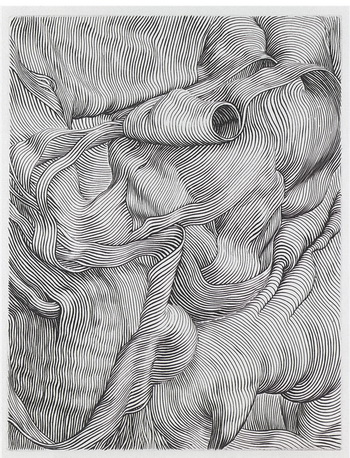The image appears to be an intricate black and white drawing that features a mesmerizing array of swirling lines and curls, resembling a chaotic but captivating display of patterns. These lines twist and turn in every direction—vertical, horizontal, and diagonal—creating an almost hypnotic effect that draws the viewer in. The entire composition resembles a mass of curly hair or possibly a slinky gone wild, with some sections appearing to form holes or openings that add to the complexity. Despite the apparent randomness and lack of a clear focal point, the lines weave together in a cohesive manner, creating a sense of unity amidst the chaos. The artwork, devoid of color, utilizes varying shades of gray, black, and white to enhance the depth and dimensionality of the curls. Each viewing offers the potential to discover new aspects and details, making it a continually engaging and fascinating piece.